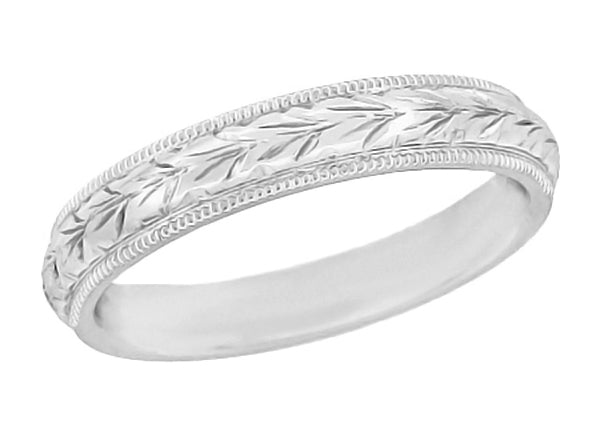The image showcases an elegant wedding band set against a plain white background. The ring, which appears to be crafted from silver, platinum, or white gold, features intricate detailing. Both the top and bottom edges of the ring are adorned with a chain or rope-like trim with jagged indentations adding texture. The central band of the ring is decorated with a continuous etching that resembles floral designs or leaves, giving an impression of delicate stems or ferns wrapping around the outer circumference. The inside of the ring is exceptionally smooth, devoid of any inscriptions or branding. The ring's positioning in the photo is slightly angled, providing a comprehensive view of its ornate, yet classic and simple design.